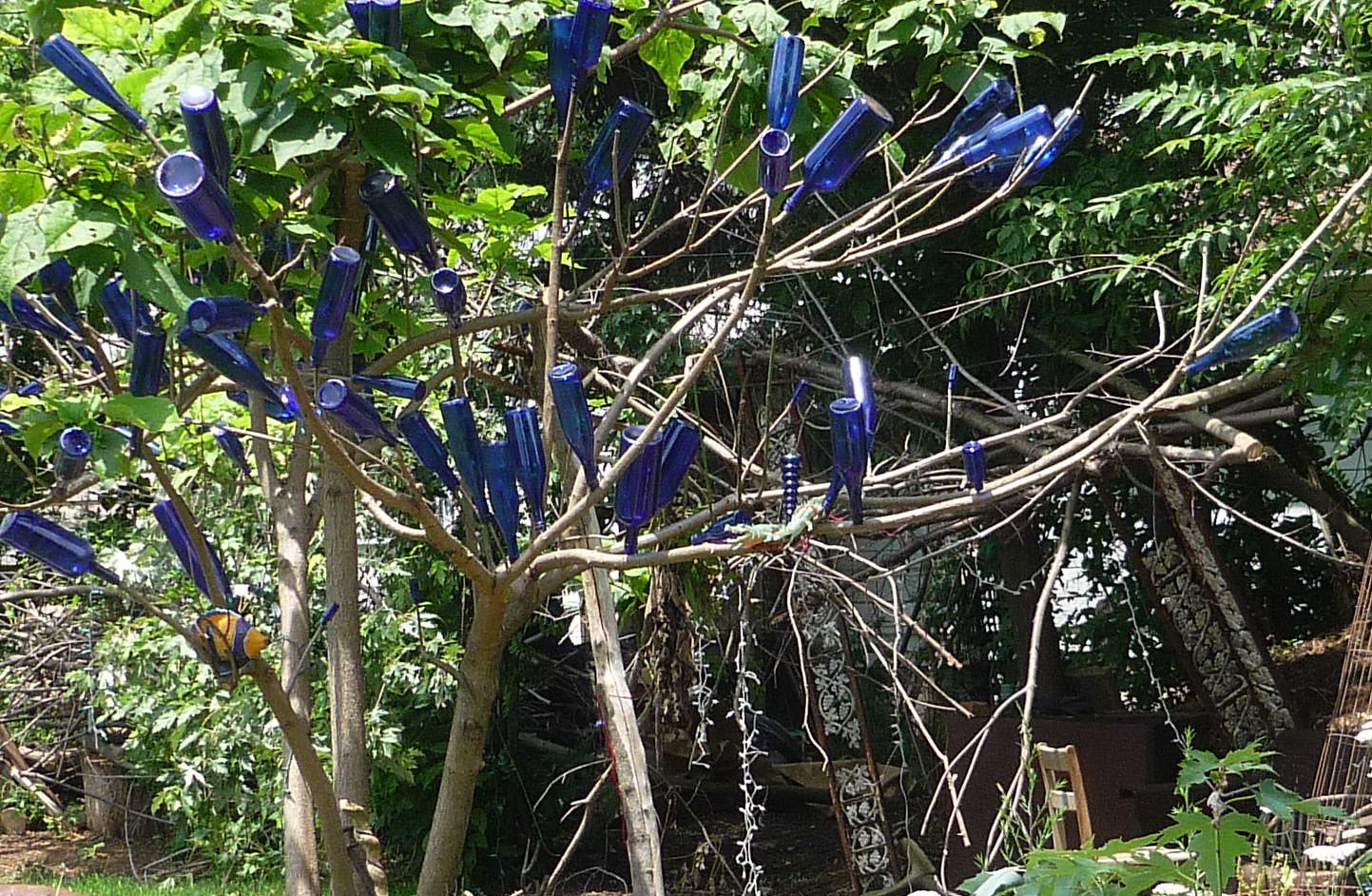This captivating outdoor photograph features a unique and artistic display of a barren tree adorned with cobalt blue bottles, which are affixed to its leafless branches, creating a striking visual effect. Each branch of the main tree hosts one or more of these blue bottles, most of which are identical in shape save for one that stands out with a rigid and slightly different design. In the backdrop, there is a picturesque arbor with intricate white filigree that adds an elegant touch to the scene. Among other details, there are verdant trees with lush green foliage behind the bottle tree, and the lower right corner reveals some indistinct wooden chairs and brown metal pieces. The blue bottles catch the sunlight, adding a shimmering quality to the image, and the entire setting exudes a blend of natural and artistic beauty.